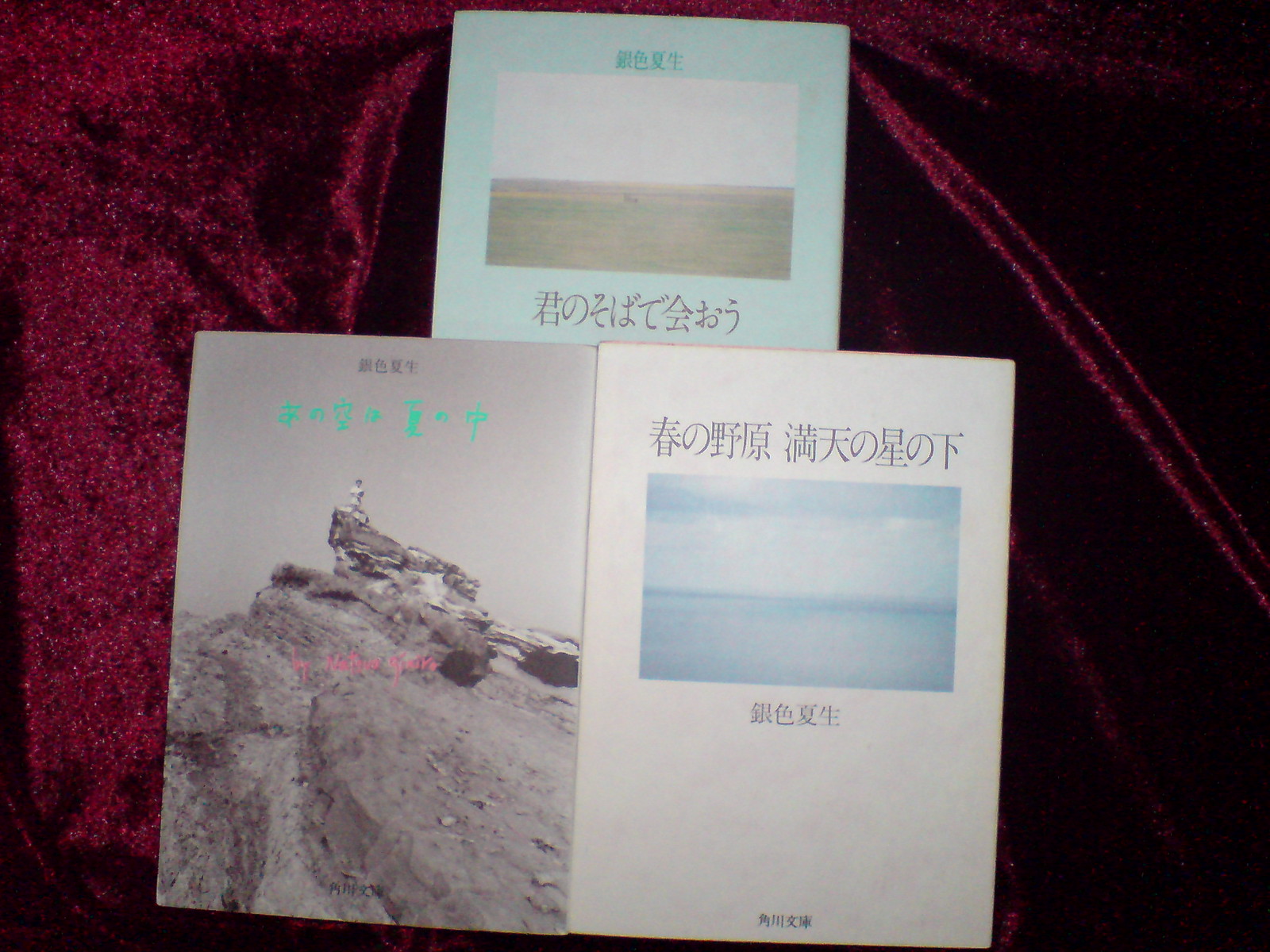The image showcases three simple-looking books, arranged on a deep, rich red velvet fabric that appears sparkly, especially in brighter areas on the left-hand side. The book at the top features a light blue cover with a photograph of an empty field or pasture, and Asian (likely Chinese or Japanese) characters in dark green at the top and black beneath the picture. Below this top book, two books are placed side by side. The book on the left, with a gray cover, shows a monochrome image of a man standing atop a rocky outcrop, with various Asian text in pink, green, and black around the image. The book on the right has a white cover with a smaller photograph depicting a seascape—a horizon of blue water and sky—encased in a rectangular frame. This book features neat black Asian characters both above and below the photograph. The entire setting is cohesive, with the three distinctive books lying on the plush, textured velvet, suggesting an intriguing contrast between the simplicity of the books and the luxurious background.